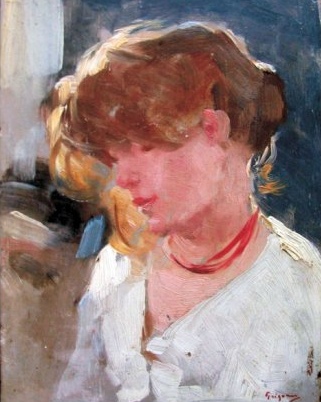This painting portrays a young woman, likely in her early to mid-20s, rendered in an impressionistic style with broad, expressive brushstrokes. She has a warm, peach complexion and reddish-brown hair that is pulled up, with strands of lighter-highlighted hair cascading around her face. Her attire includes a white blouse with a V-neck, accentuated by a red necklace that resembles a ribbon. The woman's gaze is slightly downward, with eyes obscured, as if she is deep in thought. Behind her, the scene includes muted earth tones and soft colors, featuring a grayish-blue wall, a white wall or curtain to the left, and a clay-colored floor area. The light streaming in from a window on the left softens the overall ambiance, adding to the introspective and serene mood of the portrait. Her face is the focal point, becoming less distinct as you move outward, inviting the viewer to linger on her thoughtful expression and the subtle details surrounding her.